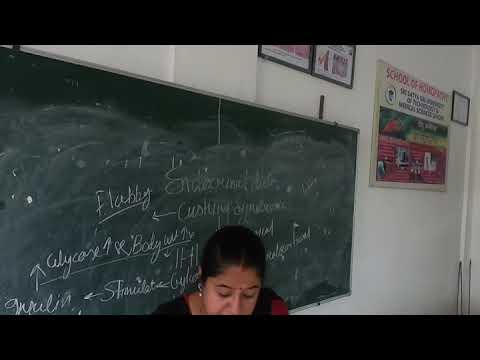The image shows a classroom interior featuring a teacher with black hair tied in a bun and silver earrings, dressed in a black and red dress. She is looking down, perhaps focusing on her lesson. Behind her, a green chalkboard is mounted on a white wall, covered with extensive white chalk writing in cursive, including words like "flabby," "blue post," and "body." To the side of the chalkboard, a sign with various graphics reads in partially legible text, "School of..." with further text in both red and black fonts. Above the chalkboard, several black-framed pictures are displayed. Notably, no students are visible within the image, highlighting the teacher and her work environment.